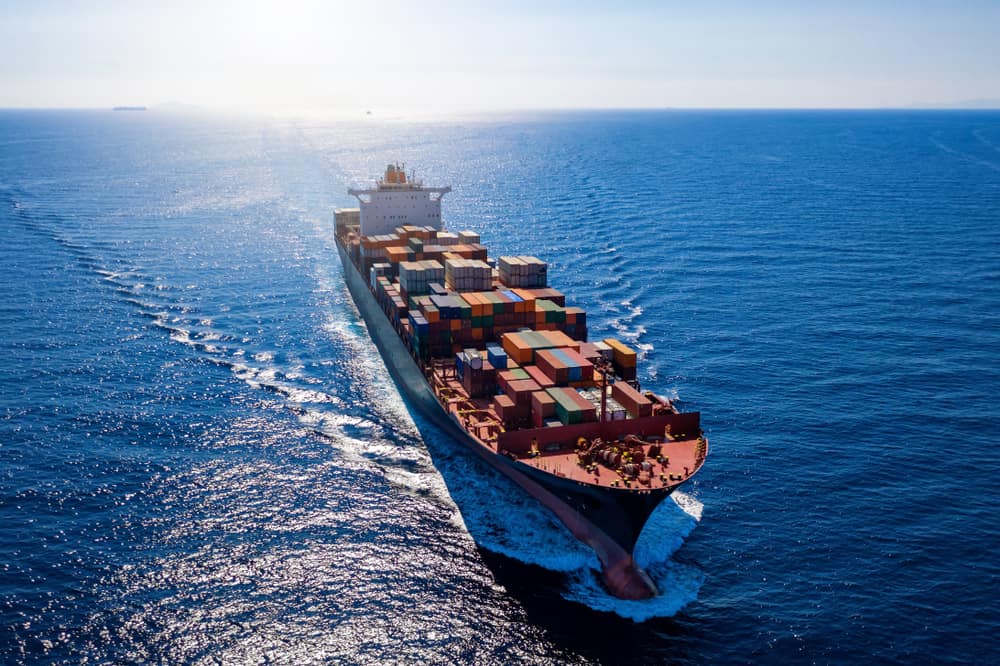The image captures a vivid photograph of a large cargo ship advancing toward the camera on the open ocean. The dark blue water contrasts strikingly with the multicolored shipping containers stacked high on the ship's deck, giving the scene an almost surreal quality. The sun, low on the horizon, bathes the containers and the ship in a warm glow, enhancing the vibrant colors. The perspective appears elevated, possibly from above, showing the full expanse from the bow to the stern, including the main cabin where the ship's captain commands. The ship leaves ripples and small waves in its wake, cutting a clear path through the calm, blue sea. The sky, clear and illuminated by the sun’s light, gives off a serene atmosphere. In the distant horizon, there is a faint silhouette of another object, likely another ship, blending into the bright sunlight. The ship's shadow stretches on the water, adding depth to this captivating, sea-adventure scene.